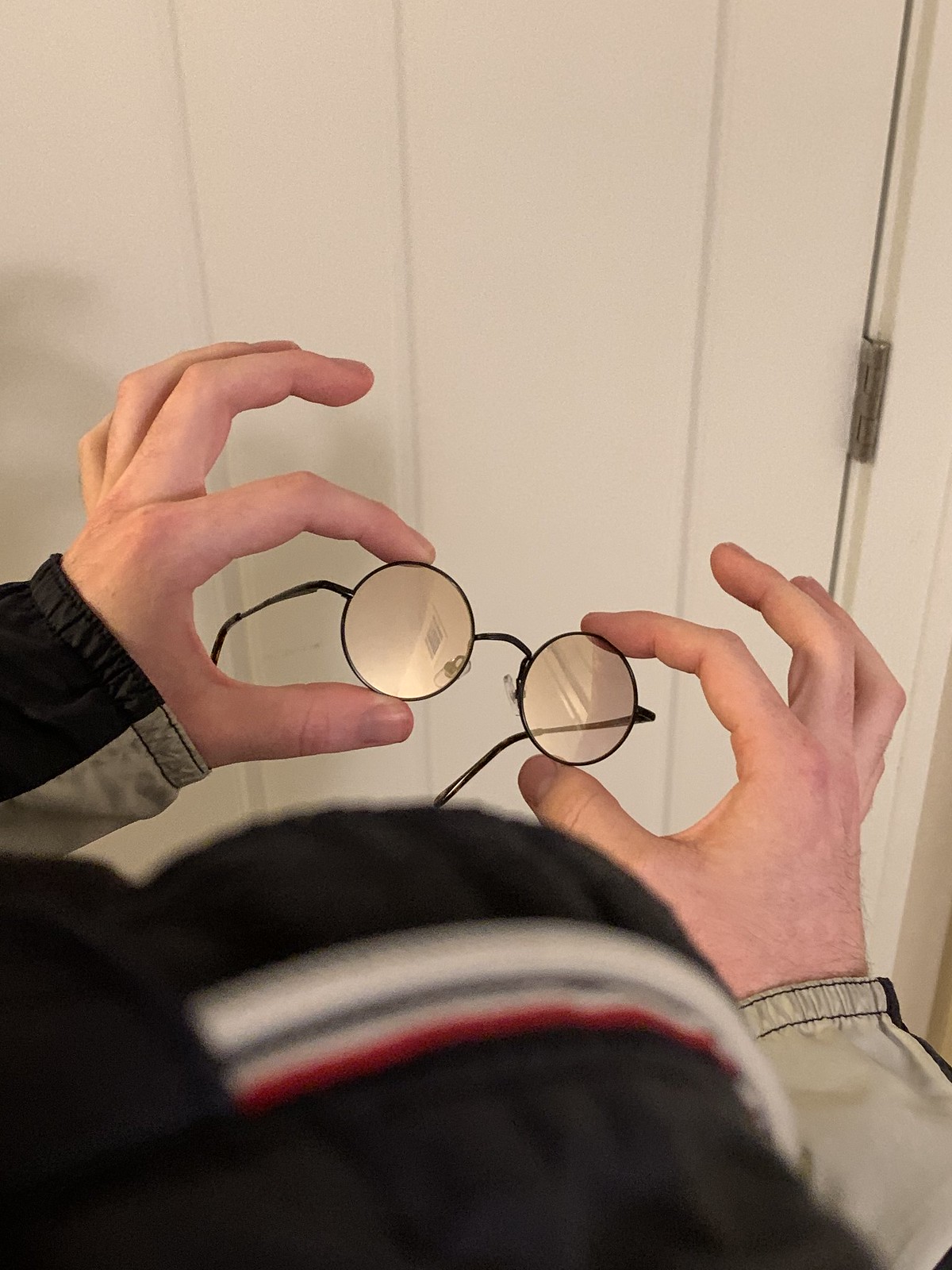This is a color photograph of a Caucasian man holding a pair of glasses, viewed from an over-the-shoulder perspective. The man, presumed to be adult, is holding his thin-framed, circular glasses with both hands, using his thumbs and index fingers. His hands are notably hairy with well-trimmed fingernails. He is wearing a jacket that primarily features black and tan colors, adorned with a stripe of white, blue, and red running down the arm, and a white zipper down the middle. The glasses have a simple, black wire frame with round lenses that appear slightly tinted or yellowish. The background shows a plain white door with vertical stripes and a brown hinge. The overall image has a slightly blurry quality, with the focus mainly on the glasses and the man's hands.